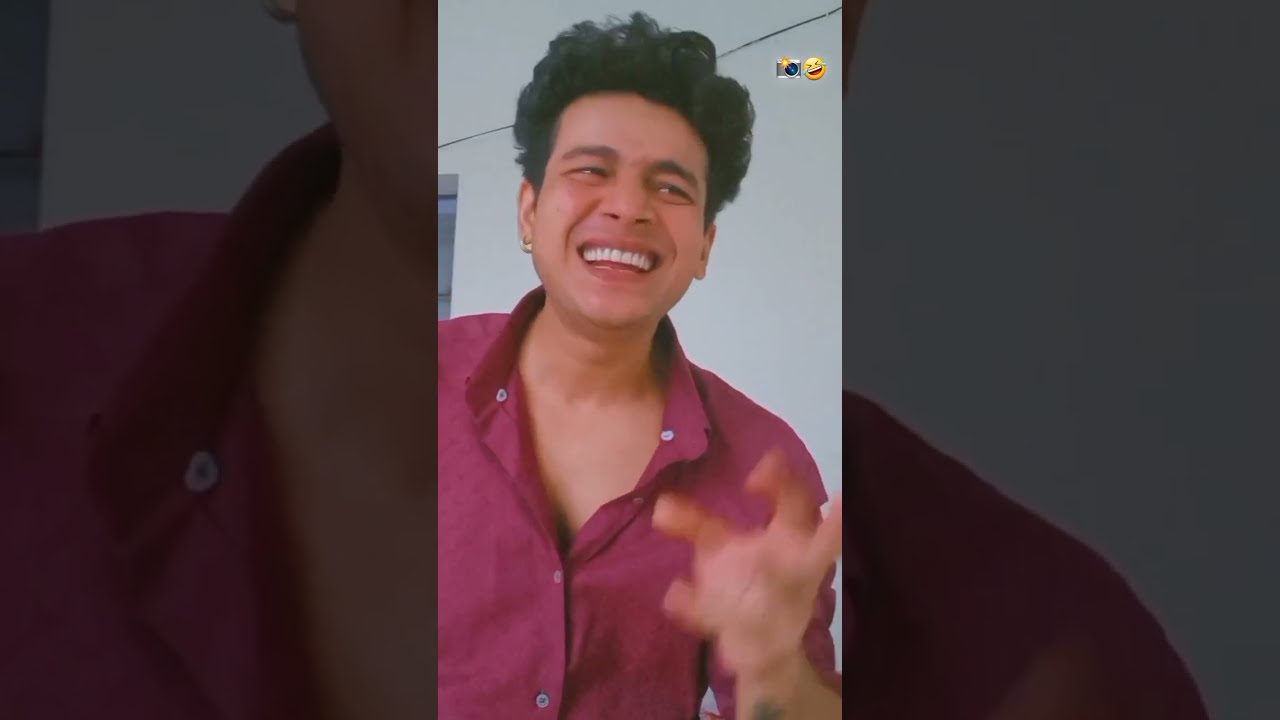This image presents a young man, possibly in his late teens or early 20s, smiling while looking towards his left. The subject has curly, bushy, dark brown hair and a mid-laugh, pained yet joyful expression, enhancing the image's humorous tone. He wears a maroon-colored button-up shirt with the first two buttons undone, partially revealing his chest. His right hand is raised, fingers in a shape reminiscent of an animal scratch. Behind him is a plain white wall. The photograph is composed of a central image and two close-up shots on either side that focus on his shirt and upper neck area. In the upper right corner, there is a crying-laughing emoji accompanied by a small silver camera icon, suggesting the photo is from a comical video, possibly a TikTok or YouTube short. The setting appears to be a home environment. Overall, the detailed elements of his expression, attire, and the accompanying visual icons highlight a light-hearted and humorous moment.